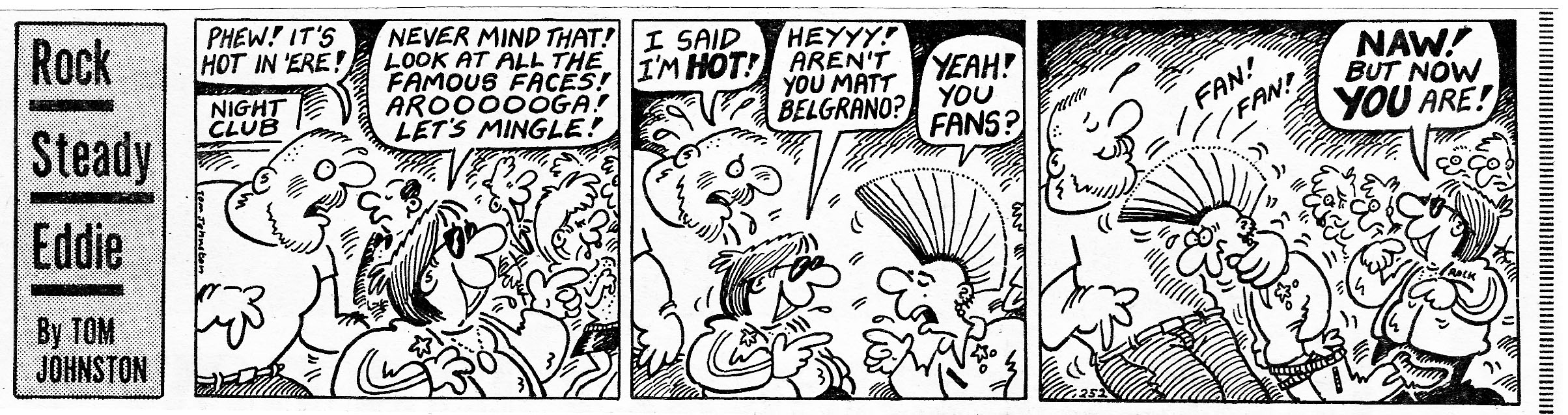This black and white comic strip, titled "Rock Steady Eddie" by Tom Johnston, is a scan, likely from a newspaper. The strip is horizontal, consisting of three rectangular panels, each depicting various scenes in a crowded nightclub. In the first panel, a man comments, "Phew, it's hot in here," while standing next to a nightclub sign. Another character, wearing sunglasses and a necklace, responds, "Never mind that. Look at all the famous faces. Aruga, let's mingle." The second panel introduces a man with a mohawk alongside the previously mentioned characters, all continuing their conversation amidst the lively club atmosphere. The third panel continues with these three characters and the bustling crowd, detailing their interactions in a humorous manner.